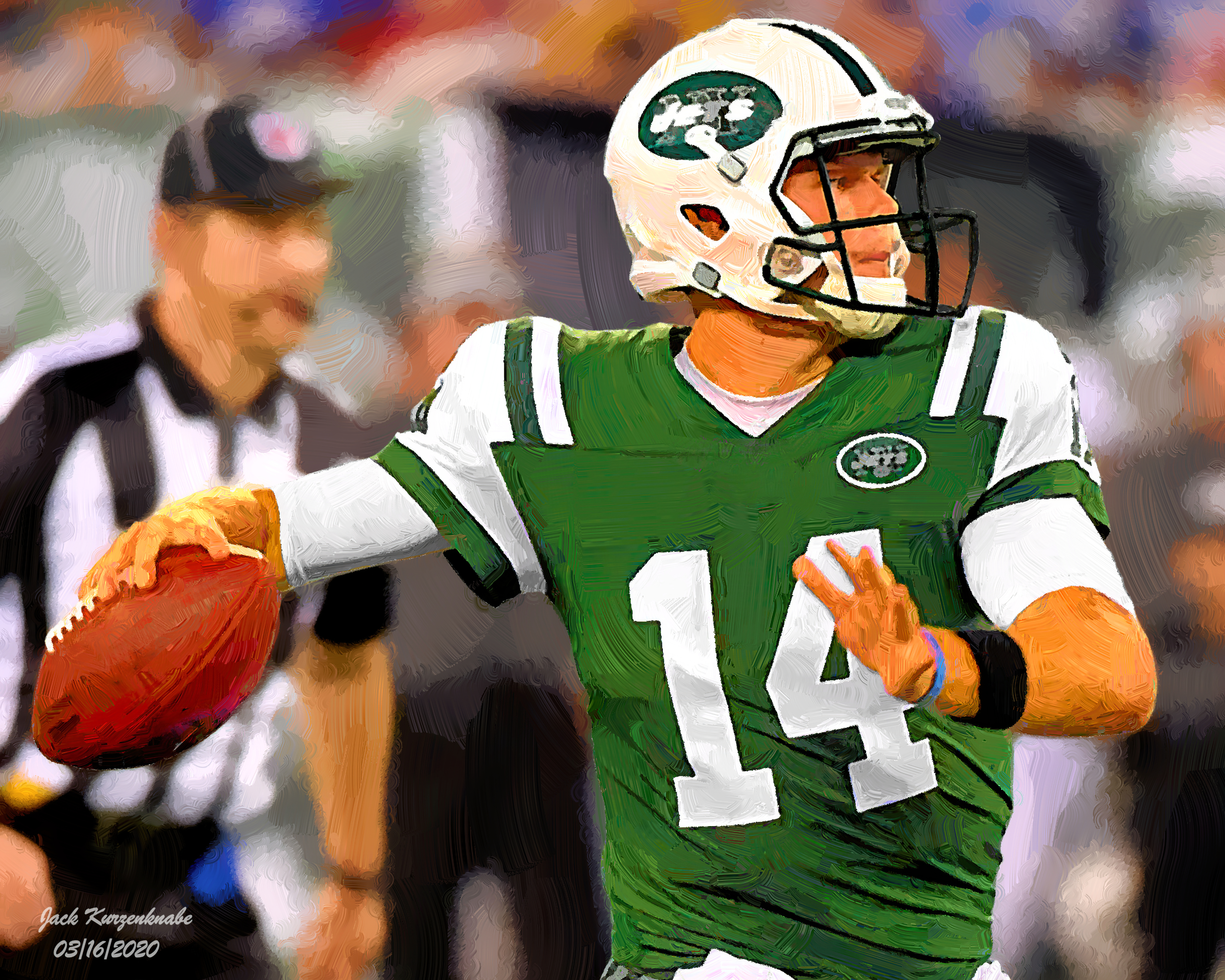This image portrays a football player rendered in a stylized, slightly cartoonish effect, wearing a green jersey adorned with white stripes and the number 14 in white. He is poised to throw a football with his right hand, his arm raised to about shoulder level, and his left elbow bent with the palm open near his chest. His uniform also features a white helmet displaying the Jets logo, complemented by a white chin guard and a black face mask. His left wrist sports a black wristband and a blue bracelet. The background, blurred for emphasis on the player, faintly shows a referee dressed in a black and white striped shirt, a black cap, and a brownish beard. The lower corner of the image contains the text, "Jack Kinganack 05-16-2020," within the almost square frame.